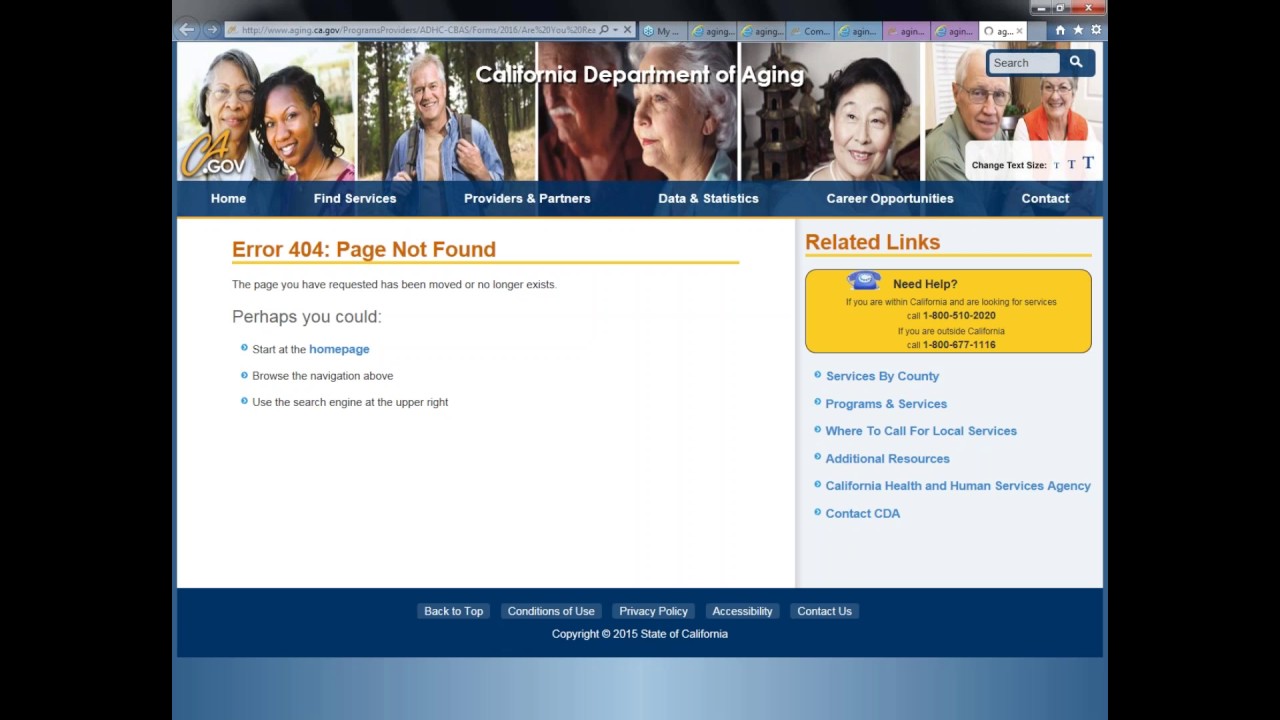In this vintage screenshot from the California Department of Aging website, the top center is prominently labeled with the agency's name. Five distinct photos are displayed beneath the header. To the left of the page, the URL "ca.gov" is visible, while on the right side, there is a search bar along with an option to adjust the text size. The navigation menu includes several clickable tabs labeled as Home, Find Services, Providers and Partners, Data and Statistics, Career Opportunities, and Contact.

Below the photos, the main content reveals an "Error 404: Page Not Found" message, indicating that the requested page has either been moved or no longer exists. Users are suggested to start at the home page, use the navigation links above, or utilize the search engine on the upper right for further assistance.

On the right side of the website, there is a "Related Links" section with a "Need Help?" prompt. If located within California and seeking services, users can contact the provided phone number. An additional phone number is available for those outside California. Several call-to-action buttons are positioned beneath this information for easy access.